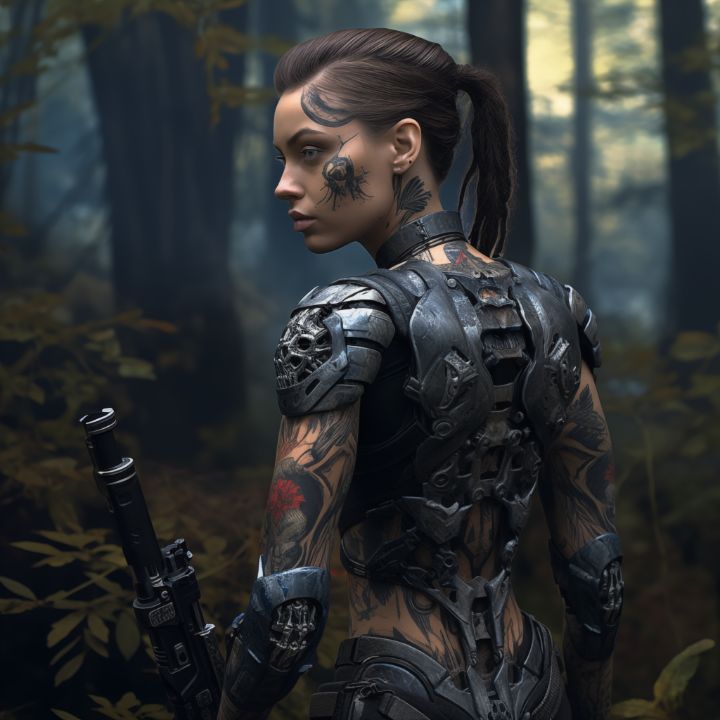In this square-shaped, digitally generated, cyberpunk-themed image, we see a heavily tattooed female character standing in a dimly lit forest during the day. The forest features brown trees with wide trunks in the background, dark green shrubbery, and a light yellow sky peeking through the foliage. The character has brown hair tied in a ponytail and light-colored skin adorned with intricate tattoos, which are primarily black but include splashes of color, such as a red rose on her left arm and a bird on her neck.

She is dressed in black metallic armor that covers her shoulders, chest, lower arms, hips, and parts of her back, with some sections revealing her tattooed skin, including her lower back and hips. The armor is detailed and futuristic, with a metal bar running up her spine, and sections protecting her elbows. 

She stands facing left, giving us a profile view of her face that highlights additional tattoos, like a spider on her left cheek and a moon on the left side of her forehead. Her stance is that of a warrior, holding a large gun in her left hand and looking off into the distance with a vigilant expression. The image combines elements of realism and graphic design, contributing to its highly stylized, almost video game-like aesthetic.